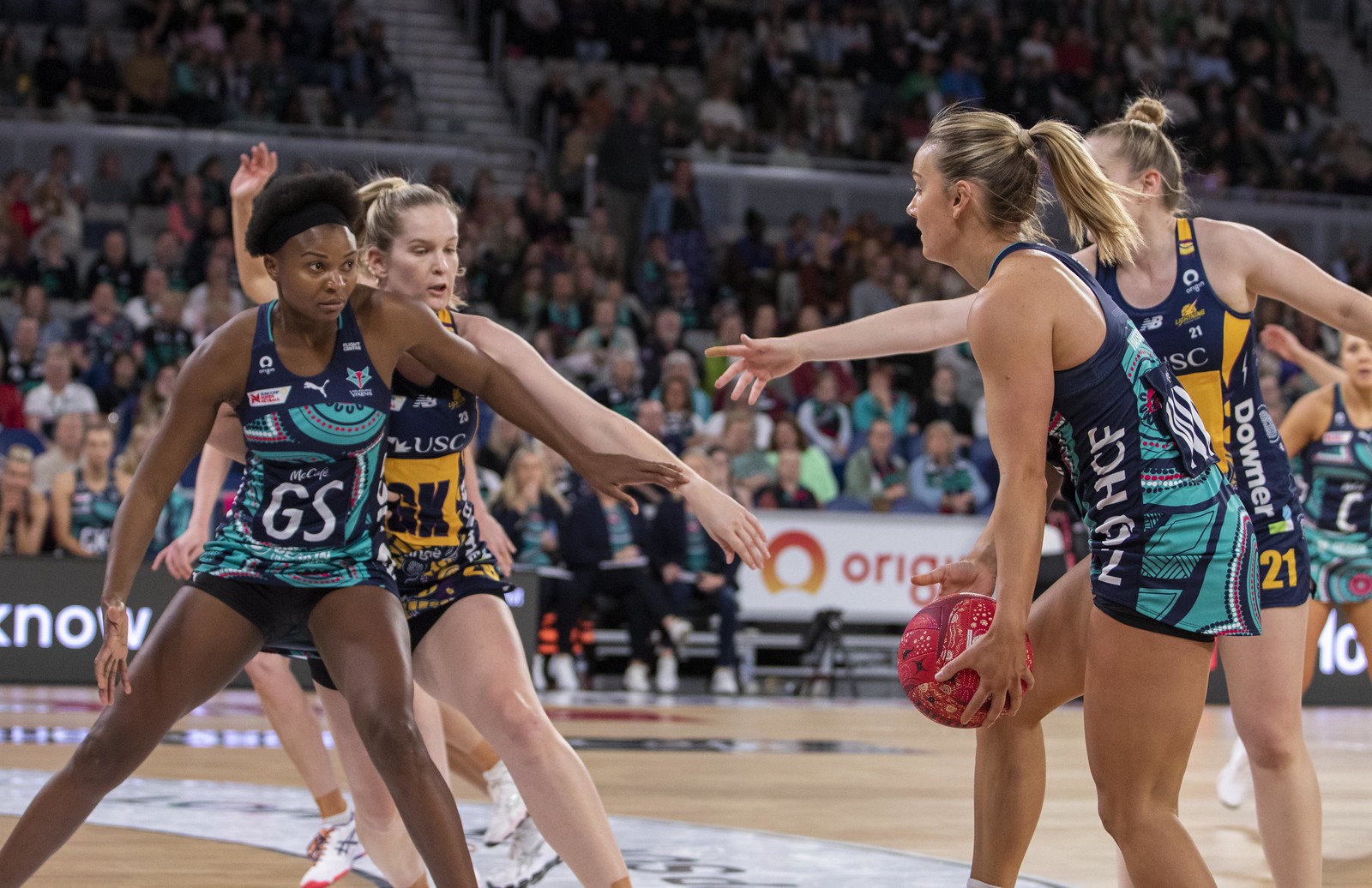This image captures an intense moment in a professional netball game, played on a polished wooden court in a bustling arena. Four players dominate the scene, with two women in the foreground and two in the background. The focal player on the right forefront, a white woman with blonde hair, is clad in a green and black (teal and dark blue) jersey and tightly grips a red netball. Positioned behind her is an opponent, also white, distinguishable by her black and yellow (or yellow and dark blue) jersey and blonde hair tied in a ponytail.

To the left, a Black woman with a green and black (teal and dark blue) jersey reaches out with her left hand, keeping her right hand at her side. She is also a teammate of the ball holder. Behind her stands another opponent, also in a black and yellow (yellow and dark blue) jersey, with blonde hair. 

The background reveals a crowded arena, with spectators filling the stands. Centrally located in the foreground, the team bench and coaches are visible with signs displayed along the base of the stands. The competitive atmosphere of the professional netball match is vividly depicted with the dynamic positions and expressions of the players.